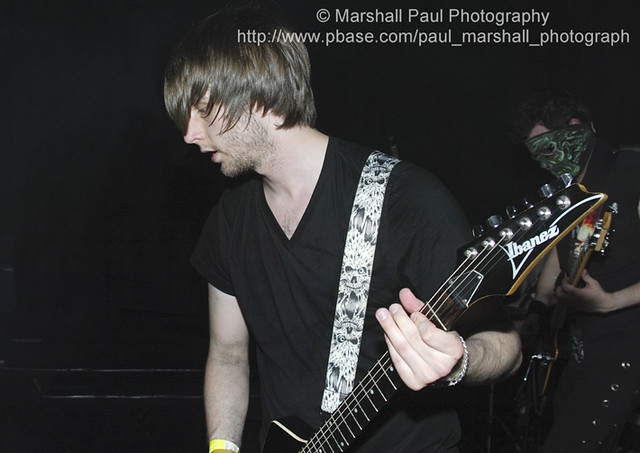In the center of this dimly-lit indoor image, a man stands prominently, holding an electric guitar with a black and white strap slung over his left shoulder. He has decently long brown hair and a slightly messy, mostly-shaved beard. He is dressed in a black shirt and sports a distinctive yellow and white wristband on one hand, with a silver bracelet on the other, which is gripping the guitar's neck. The guitar itself is detailed with black, white, and brown elements, including silver knobs and strings, and has "Ibanez" inscribed on it. Behind him stands another man, partially obscured by shadows, wearing a black shirt and a green and black mask. This second man is also holding a guitar. The ambient darkness of the room suggests an intimate setting, perhaps during a band rehearsal. The top right corner of the image features a watermark stating "Copyright Marshall Paul Photography" alongside the URL "pbase.com/PaulMarshallPhotograph." The image's color palette includes black, white, tan, brown, gray, red, orange, yellow, and green.